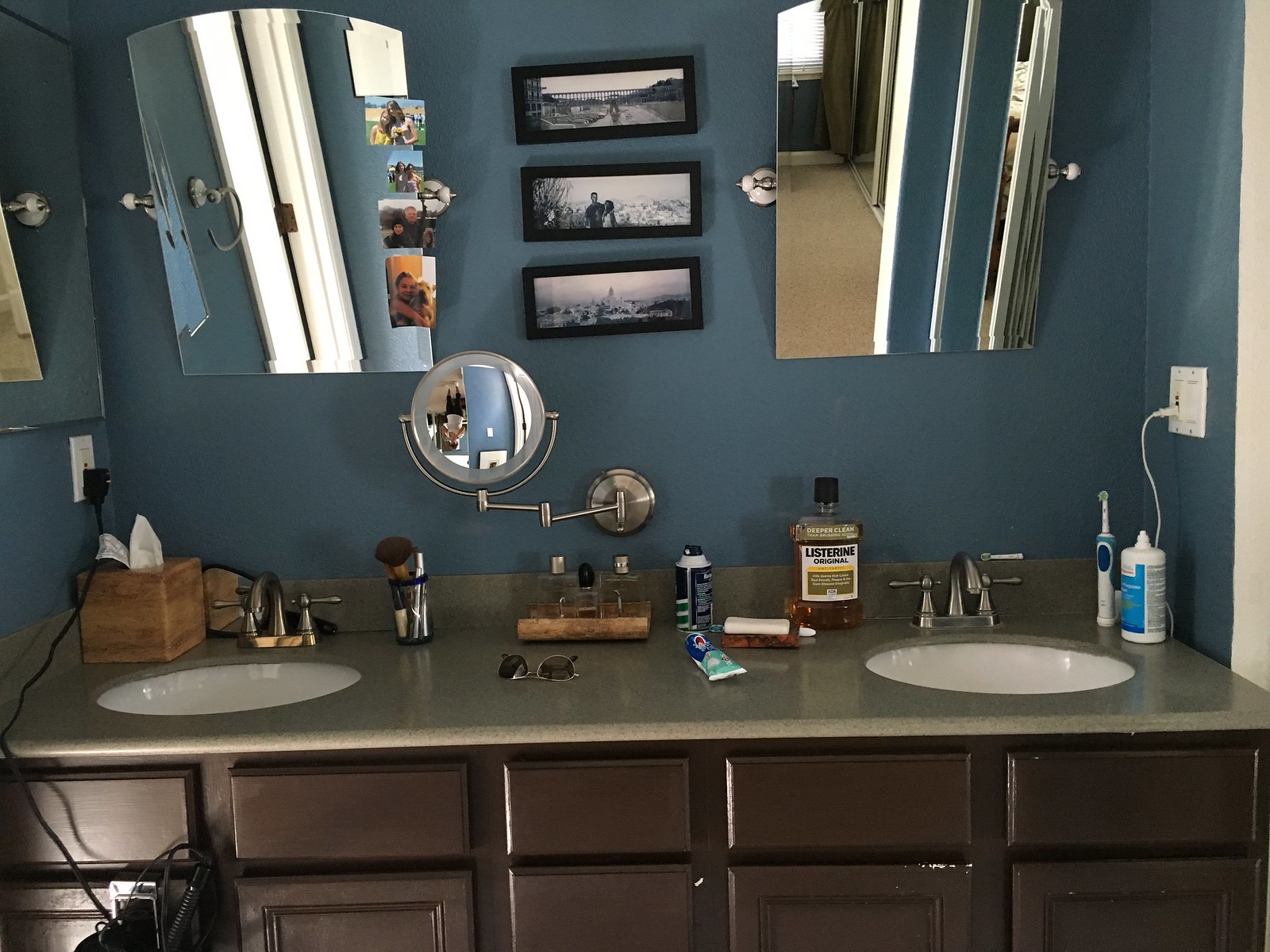This photo captures a meticulously arranged bathroom with dual sinks and a combination of modern and personal touches. Each sink is topped with a large, equally sized mirror. The mirror on the left is accessorized with several small photos affixed to its right edge, adding a personal flair. Trio of framed black-and-white photographs are symmetrically placed between the two mirrors, balancing the decor. Just beneath these framed pictures, a circular magnifying mirror is attached to the wall, providing practical convenience.

The countertop is well-organized and functional: starting from the left, a tissue box is situated next to the first sink, followed by a small container filled with makeup brushes, and another small container for colognes. A pair of sunglasses rests casually next to a can of shaving cream and a tube of Crest toothpaste. Near the bar of soap, there is a plastic jar of original Listerine, placed just before the second sink. On the other side of this sink, an electric toothbrush and a plastic jar of contact lens solution complete the countertop arrangement.

Electrical outlets are conveniently located on either side of the sinks, above a set of dark wood drawers and cabinets that provide ample storage. The wall above the sinks is painted a calming grayish blue, adding a serene backdrop to the room's functionality.